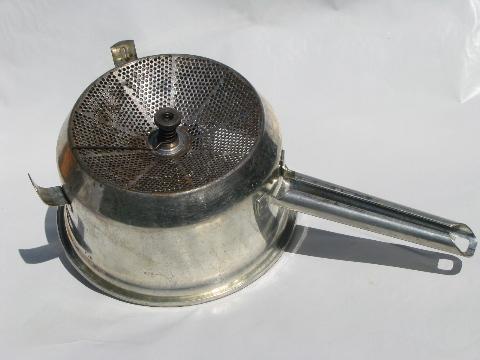The image depicts a horizontally aligned rectangular photograph showcasing an old and worn kitchen sifter set against a white, slightly marbled countertop. The sifter features a rounded stainless steel body with a fine mesh design and a concave vented lid that has a rusted screw in the center. The right side of the sifter has a dull, cylindrical handle with visible rust marks, indicating it needs cleaning. On either side of the sifter are small metal pieces, likely hooks for securing or hanging over a pot or bowl. The overall appearance suggests it is used for sprinkling powdered ingredients, such as sugar, over food. The background is a light white surface, enhancing the contrast with the aged, silver kitchen tool.